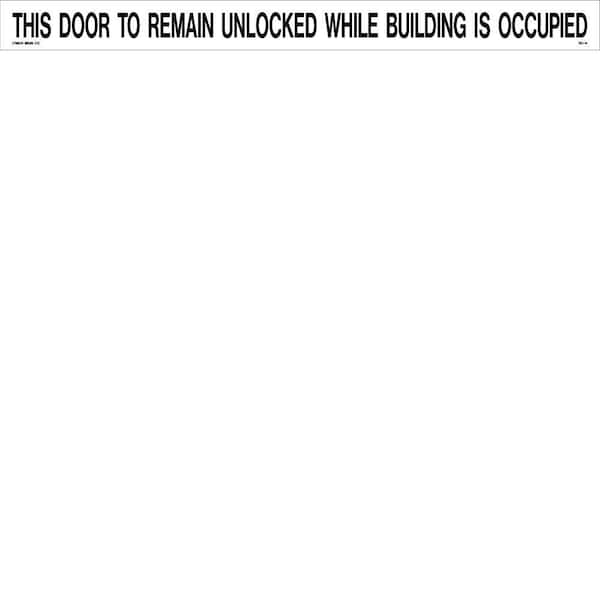The image depicts a rectangular sign designed to provide important information. The central focus of the sign is the text displayed in large, black capital letters against a white background, which ensures high visibility and readability. This sign is bordered by a thin, dark gray line, neatly framing the text and adding a subtle yet effective emphasis. The message on the sign reads: "THIS DOOR TO REMAIN UNLOCKED WHILE BUILDING IS OCCUPIED." This clear and concise directive indicates that the sign is intended for placement inside a building, specifically above exit doors, to ensure compliance with safety regulations. There are no additional elements or distractions in the image; it solely features the sign and its essential message.